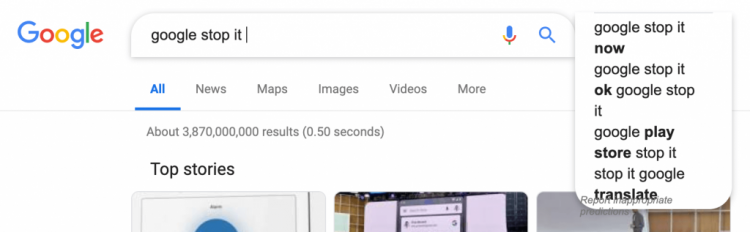This Google search results page showcases the query “Google Stop It” at the top. The search bar prominently displays the query along with a blue microphone icon and a blue magnifying glass icon for voice and manual search options. On the right-hand side of the page, related searches are listed including “Google Stop It Now,” “Google Stop It,” “OK Google, Stop It,” “Google Play Store Stop It,” and “Stop It Google Translate.” 

The results are divided into various sections, with the ‘All’ tab highlighted in blue, indicating the active section. Other available options for filtering results include ‘News,’ ‘Maps,’ ‘Images,’ ‘Videos,’ and ‘More,’ each label written in gray text beneath the multicolored Google logo.

The 'Top Stories' section is also present, featuring a selection of partial images and headlines: one appears to show a blue circular element with text, another might depict a smartphone screen or stage set against a white background, and a third possibly illustrates an outdoor billboard with a white backdrop and a wooden-paneled wall. Black text accompanies these image thumbnails, adding context to the search results.